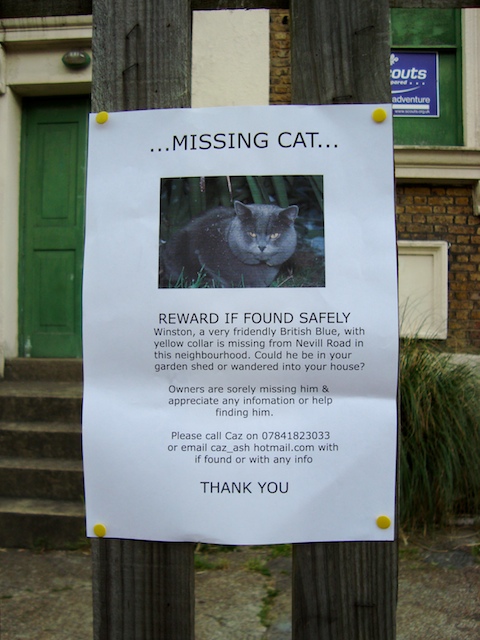The image shows a detailed outdoor photograph of a missing cat notice pinned to two vertical wooden poles using four yellow pins, one at each corner. At the top of the poster, in bold black letters, it reads "Missing Cat". Directly below is a picture of Winston, a dark grey British Blue with yellow eyes wearing a yellow collar. The notice continues with, "Reward if found safely," and provides the details: Winston is a very friendly British Blue who has gone missing from Neville Road in this neighborhood. The poster questions if Winston could be in someone's garden shed or house and emphasizes that his owners are sorely missing him and would be grateful for any help or information about his whereabouts. Contact details are provided as follows: please call CAS at 0784-182-3033 or email cas_ash at hotmail.com with any information. Thank you. In the background, there are additional details of the surrounding area, including brick walls, a house with steps leading up to a green door, white plastered walls, and a sidewalk.